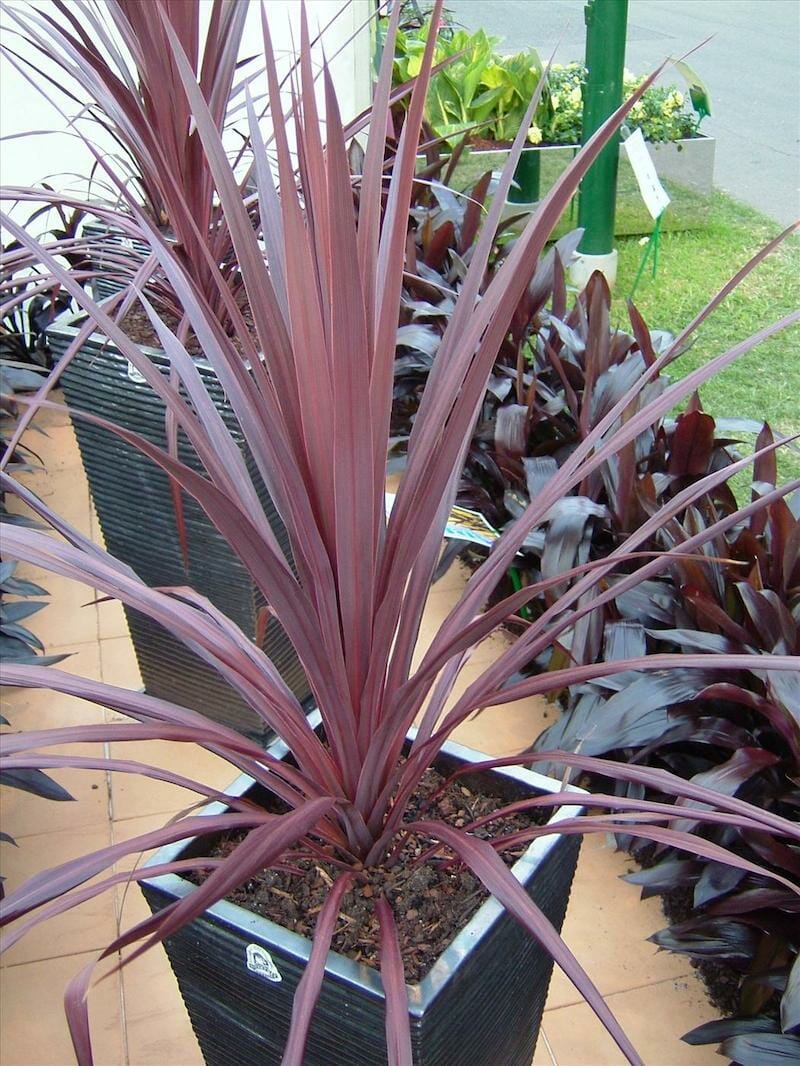The close-up image captures a potted plant with long, spiky, rose-colored leaves that are reminiscent of palm leaves. The leaves emerge from a large, dark greenish-black square ceramic planter with horizontal grooves. The pot reveals the topsoil, highlighting the plant's grounding. In the background stands another, taller planter with a similar plant, partially obscured by the angle of the photo. Surrounding the focal plant are rows of larger leaves growing directly from the ground, their blackish-reddish hue adding to the scene's vivid palette. These rows frame the patio, which is laid with light-colored tan tiles. On the right, a stainless steel planter box full of green plants and flowers reflects the adjacent grass and a green pole, adding depth to the image. A glimpse of a road in the upper right corner completes the scene, weaving elements of nature and structure seamlessly together.